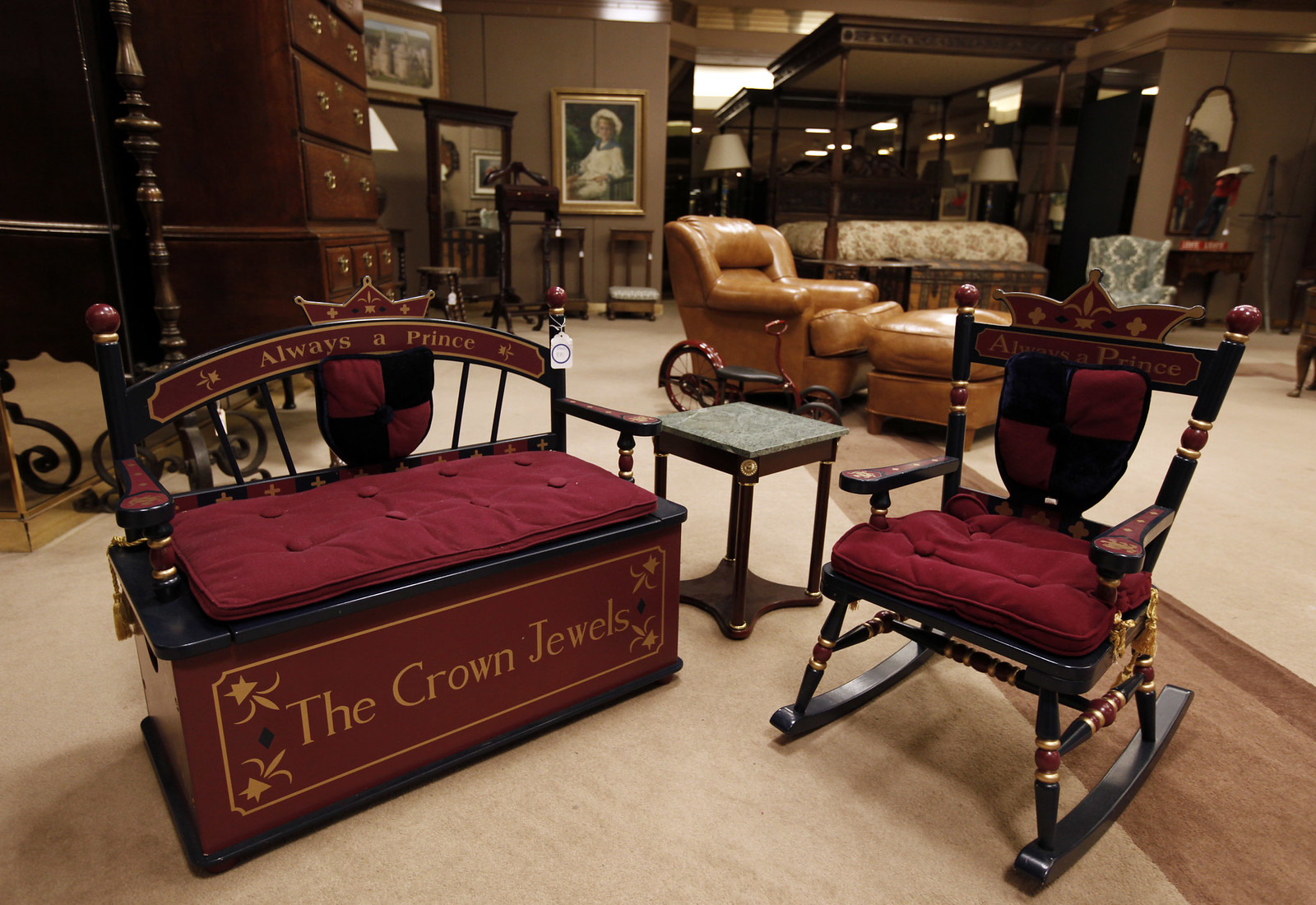The image appears to be taken in a well-decorated showroom, likely designed to display antique or vintage-style furniture, possibly for sale given the presence of tags on the items. The room has a Victorian or French palace aesthetic, with rich wooden furniture and various accessories. On the left side, there is a small, black and red toddler seat with red cushions, a crown-shaped decoration above the backrest, and inscriptions reading "The Crown Jewels" at the bottom and "Always a Prince" at the top. Adjacent to this is a matching rocking chair with similar inscriptions and design features, including a small crown and the phrase "Always a Prince" at the top. Between the two seats stands a tiny end table. The background showcases a large wooden dresser, an ornate wooden mirror, and several paintings. A four-poster bed with an overhang occupies the center, accompanied by brown leather chairs and a footstool, adding to the room's luxurious ambiance. The overall setup, filled with various vintage furnishings and mirrors, suggests this is a meticulously arranged display area, possibly within a museum or an upscale furniture store.